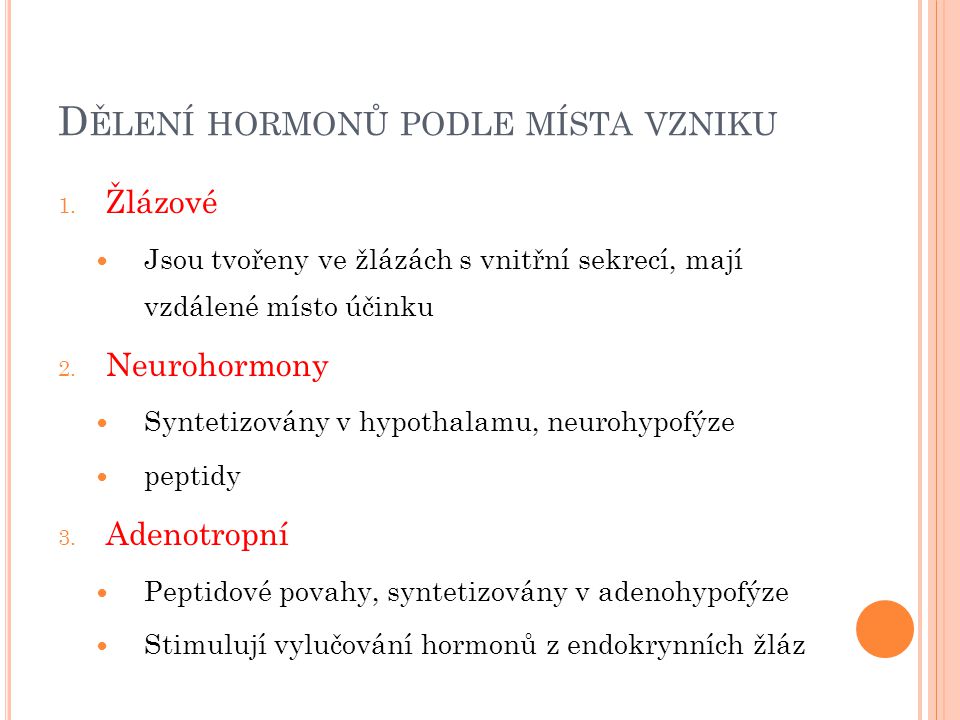This image depicts a page from a book or article, written in a foreign language. The page is bordered by lines, with a thin pinkish line running along the left edge and a thicker, reddish-orange line along the right edge. The title, comprised of five words, reads "Deleni, Hormonu, Podol, Mista, Vazniku". Below the title, the content is organized with red, bold words accompanying numbers 1, 2, and 3. Each numbered section includes bullet points—one bullet point for number 1, two bullet points for number 2, and two bullet points for number 3—each featuring additional explanatory text. The overall color scheme includes white, red, pink, and orange, with a notable round orange circle positioned at the bottom right corner of the page.